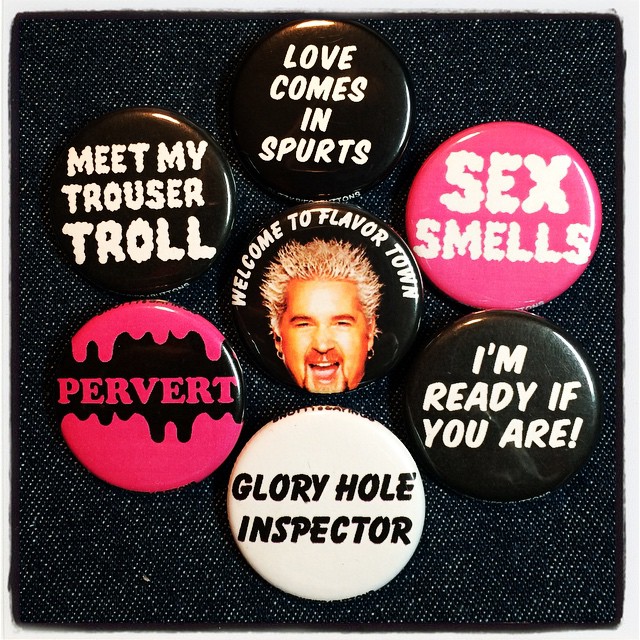The image showcases a collection of seven metal pins arranged on a black denim background. At the center is an eye-catching pin featuring a vibrant portrait of Guy Fieri with his signature spiky blonde hair, smiling widely. The pin is emblazoned with the phrase "Welcome to Flavortown." Surrounding this central pin, in a clockwise arrangement, are several other pins with bold statements: "Love comes in spurts" in white letters on a black background, a hot pink pin with white cloudy font reading "Sex smells," another black pin with white text stating "I’m ready if you are," a white pin with black letters saying "Glory Hole Inspector," a black pin with pink letters spelling "Pervert," and a final black pin with white text declaring "Meet My Trouser Troll." These pins collectively create a vibrant and cheeky display on the nearly black denim square, drawing attention with their colorful and provocative messaging.